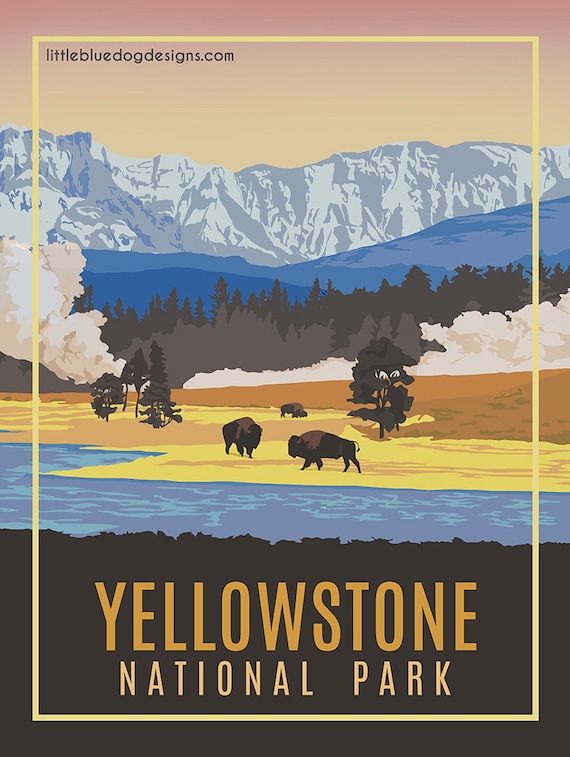This is a poster of an animated or painted graphic design depicting Yellowstone National Park, which is written in large yellow letters at the bottom of the image. The design, crafted by LittleBlueDogDesigns.com (noted in the top left corner), exhibits a richly detailed landscape from top to bottom. 

At the top, the sky transitions from pink to off-white hues, setting a tranquil tone. Below this, a majestic mountain range shifts from white and gray to a deep blue further down. Below the mountains, a dense forest of brown and black trees emerges. 

Prominently in the middle of the image, a plume of white smoke rises from the forest, adding a dynamic element to the scene. The land carries an orangish to yellowish gradient, portraying a grassy or earthy terrain. On this land, five sparse trees and three grazing bison add life to the scene, emphasizing the park's natural beauty.

Towards the lower portion of the image, a blue waterway or river snakes through the terrain, contrasting with the dark brown or light black land below it. All these elements are framed by a thin off-white border, encapsulating the design perfectly.